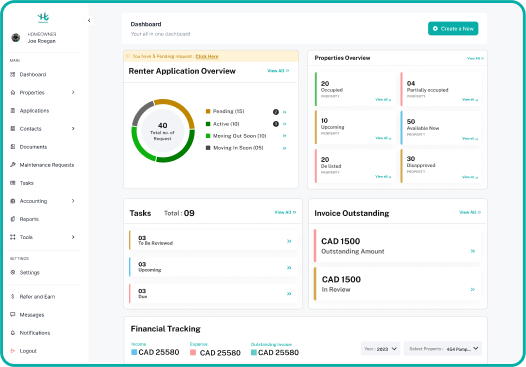**Detailed Caption:**

This screen capture showcases a financial website with a predominantly white and light gray background, outlined in turquoise blue. In the top left corner, there is a blue "H" logo, with text beneath it too small to read. Below the logo, it says "Homeowner Joe Rogan" in black, accompanied by a gray dot to the left. On the left-hand side, there is a vertical menu bar with various labels, though some are blurry. The labels from top to bottom include: Dashboard, Properties, Appliances, Contacts, an unreadable label, Maintenance Requests, Task Accounting, Reports, Tools, Settings, Refer and Earn, and Notifications. Notably, Log Out is the last, clearly visible option.

To the right of this vertical menu is an off-gray area. At the top right of this section, a turquoise bar with white lettering mentions "Dashboard" in black on the upper left. On the left side of this central area, there's a circular graphic comprised of dark green, light green, gray, and yellow segments. The top yellow segment is labeled "Eligible." This graphic is part of a "Renter Application Overview," which, on the right side, uses icons to denote statuses such as pending, active, moving out soon, and moving in soon.

To the right, the "Properties Overview" section displays property statuses in two columns per line across three lines. The statistics include: 20 properties occupied, 4 partially occupied, 10 upcoming, 50 available now, 20 delisted, and 30 disapproved.

Below this overview section lies another white section consisting of two boxes. The left box, labeled "Task," states that there are a total of 9 tasks, with a "View All" link in the upper right corner. It features three rows with black text on the left and blue arrows on the right. The right box, titled "Invoice Outstanding" in bold black, also has a "View All" link in blue on the right. It lists two rows: the first marked by a red line on the left, indicating a CAD 1500 outstanding amount, and a blue star on the right. The second row, marked by a mustard yellow-brown bar, mentions a CAD 1500 amount in review, again accompanied by a blue star on the right.

At the bottom of the page, a long white rectangular bar titled "Financial Tracking" displays various amounts in Canadian dollars. It features a blue icon to the left of the first amount, a pink icon in the center, and another blue icon for the final amount.